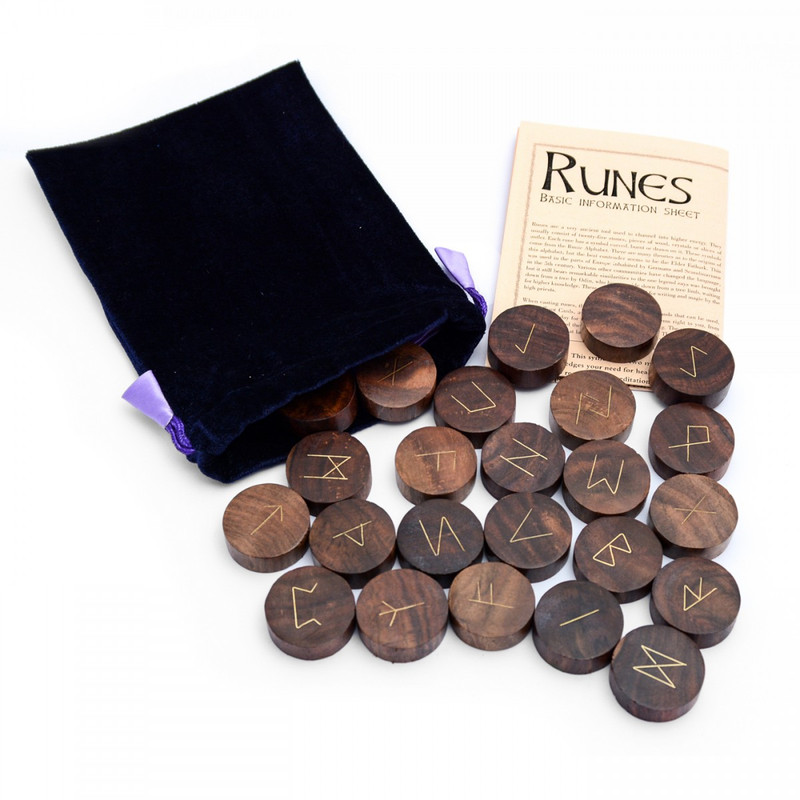**A photograph captures a set of wooden runes scattered across a white backdrop, originating from a black velvet drawstring bag equipped with purple or periwinkle ties. Some runes remain partially spilled out from the bag. The runes are round wooden discs, varying in shades from dark to medium wood, and bear engravings of ancient symbols and letters. These intricate symbols include shapes resembling S's, F's, interconnected triangles, simplified fish forms, arrows, staple-like figures, and an M with downward edges. Accompanying the runes is a pale pink folded paper labeled 'Basic Information Sheet,' providing paragraphs that explain the usage and specifics of the runes. The image highlights the intriguing blend of ancient text and modern curiosity.**